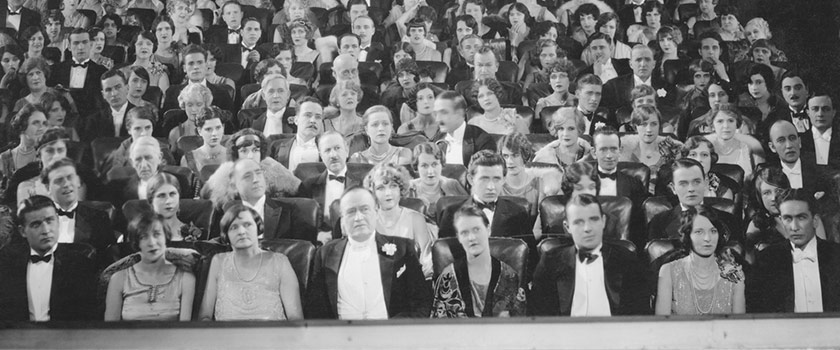This black and white photograph captures an elegant, meticulously dressed audience in a theater, with an image orientation that is a wide horizontal rectangle, approximately two and a half times wider than it is tall. The photo is taken from the stage, looking out toward the spectators. The theater seating rises upward, revealing around ten rows of individuals, all of whom are adults with a diverse age range from younger to older adults. The men in the photograph sport black tuxedos with white shirts and dark bow ties; some are accessorized with handkerchiefs or flowers on their lapels. The women display formal attire, often featuring dresses with exposed arms and styled, curly hair, accessorized with corsages. The sophisticated attire and hairstyles strongly suggest that the photo dates back to the 1920s or 1930s. The sense of wealth and status emanates from their polished appearance and the grandeur of the occasion depicted.